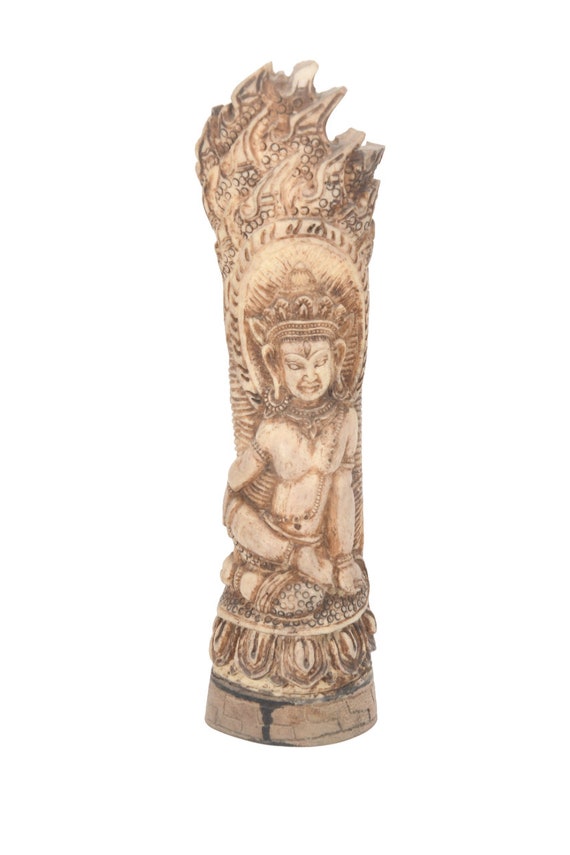This image depicts a detailed close-up of an ancient artifact, resembling a wooden totem or carved statue with origins likely from Southeast Asia or India. The totem, shaped somewhat like a torch or a vase, is intricately carved and made from a tannish material, possibly wood or ivory. Dominating the center of the carving is a deity, who appears to be a Hindu god. This figure has distinct features, including large, round earrings, a headdress with an oval shape and flames emerging from the top, representing enlightenment or spiritual attainment. The deity has a small nose, thicker lips, and a crown with a sun above its head, possibly indicating radiance or divine status.

The deity is depicted sitting cross-legged, reminiscent of a meditative or traditional Indian pose, on an inscribed seat or rug. It is shirtless, adorned with bracers on both arms, and wears multiple strings of jewelry around its neck and chest, suggesting wealth or importance. The engraving beneath the deity includes small, detailed circles and various inscriptions, but no writing. The cylindrical structure of the totem tapers downwards, featuring further engravings and black ink seeping through brick-like patterns towards the base. 

The entire carving, with its delicate yet intricate etchings and emphasis on the deity's adornments, gives off an aura of ancient religious significance and artistic craftsmanship.